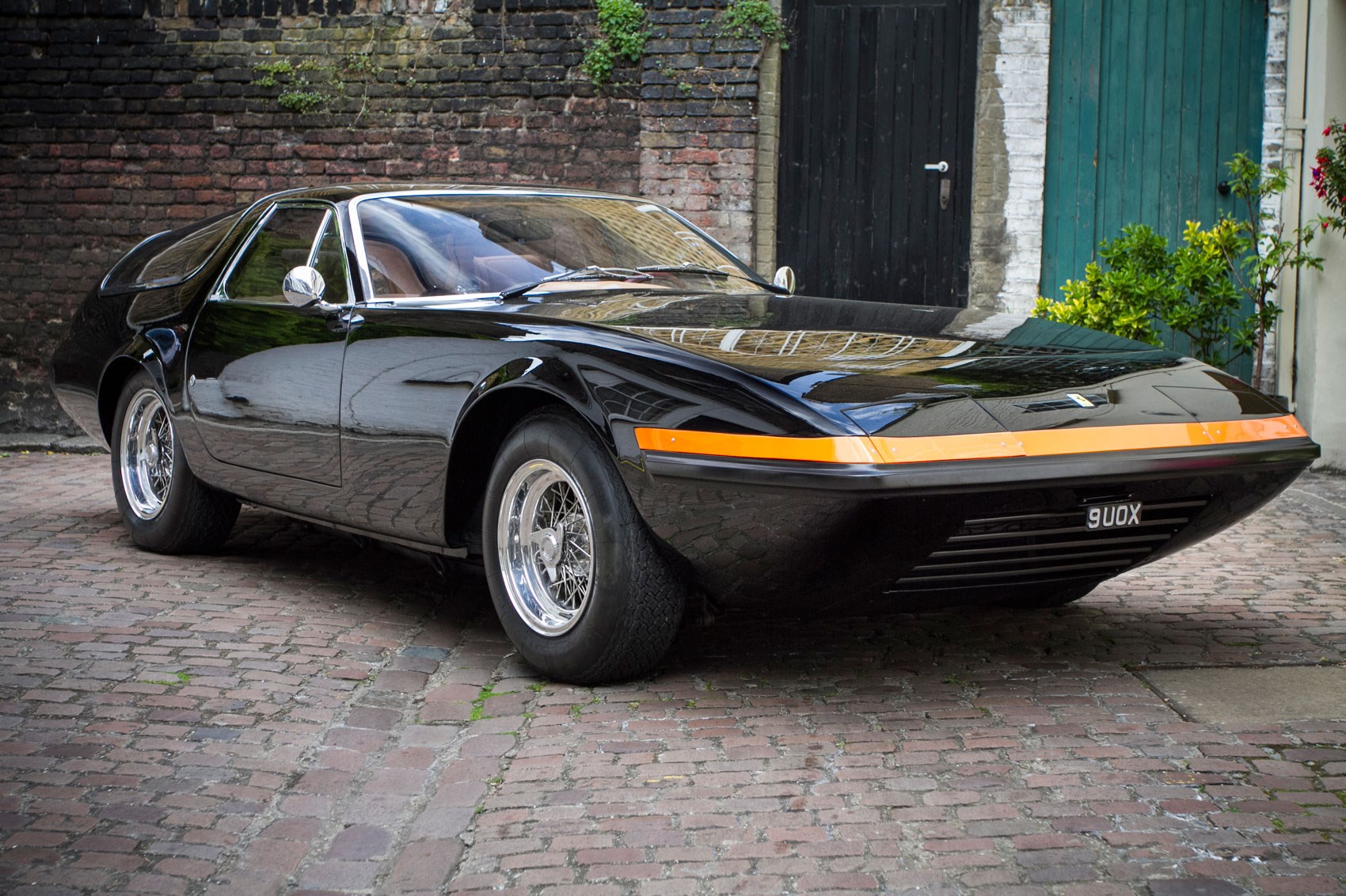This image captures a close-up of a sleek, black sports car, parked on a cobblestone driveway with varying shades of light red and brown stones. The car, facing slightly to the right, reveals its right side and front. It features a long front end with a vivid orange stripe extending from the front right tire across the front grill area, which also showcases a white license plate that reads "9UOX." The shiny, silver rims and small tires add to its luxurious appearance, along with chrome side mirrors and a likely black spoiler subtly visible at the back. The car is a two-door coupe with a large front windshield.

In the background, a weathered brick wall occupies the left side up to halfway of the image, with some greenery sprouting through it. To the right of this wall, there is a black wooden panel door with a silver handle. Further right, a partially white-painted brick column transitions into another section featuring a teal wooden wall slightly concealed by plants, adding a touch of color and natural beauty to the scene.